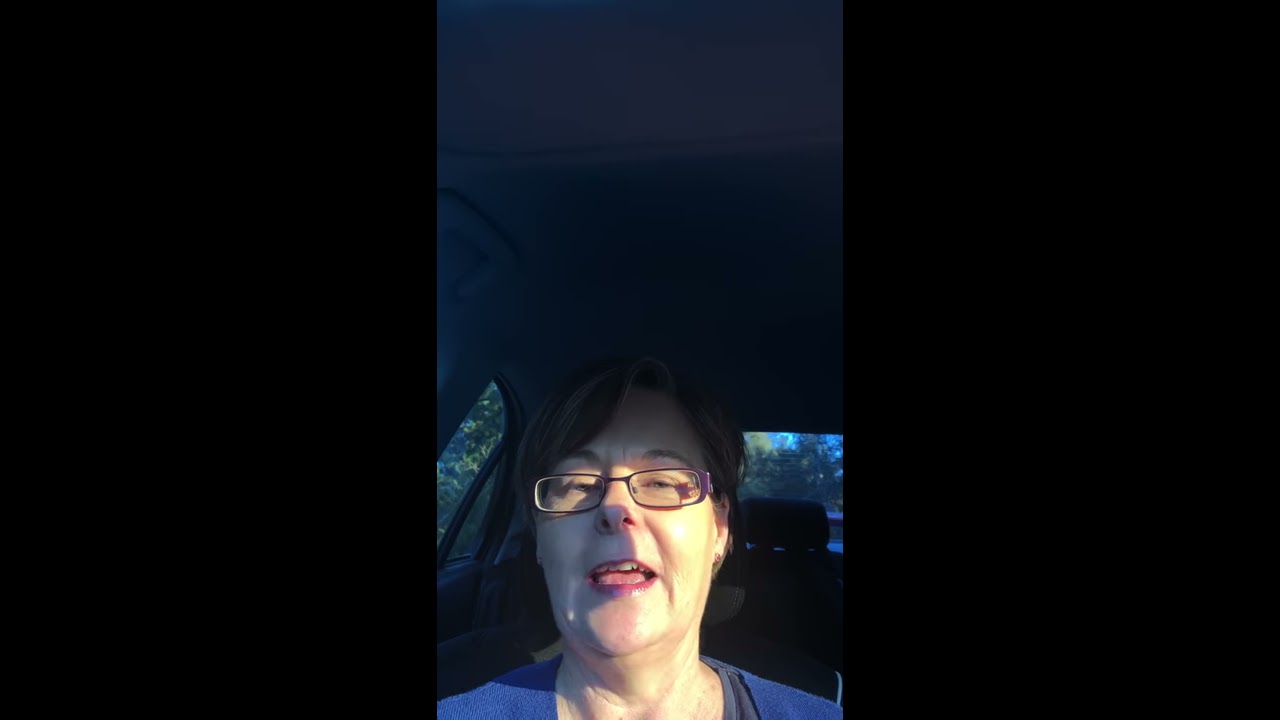A selfie of an older Caucasian woman in her 50s captures her seated in the passenger side of a car, with only the right side of her face illuminated by a subtle light. The rest of the image is enveloped in shadows, enhanced by a thick black border on the left and right-hand sides. Her brown hair, parted at the side of her bangs, is contrasted by her striking red lipstick. She dons glasses with a distinctive purple frame and studded earrings in both ears. Wearing a blue t-shirt, she appears to be speaking, her mouth partially open, displaying her top row of teeth and tongue. The car’s dark grey interior is discernible, with a handle situated just above her head on the ceiling. An empty grey seat with a headrest is visible in the back, and through the rear windows, hints of a road and lush vegetation can be seen.